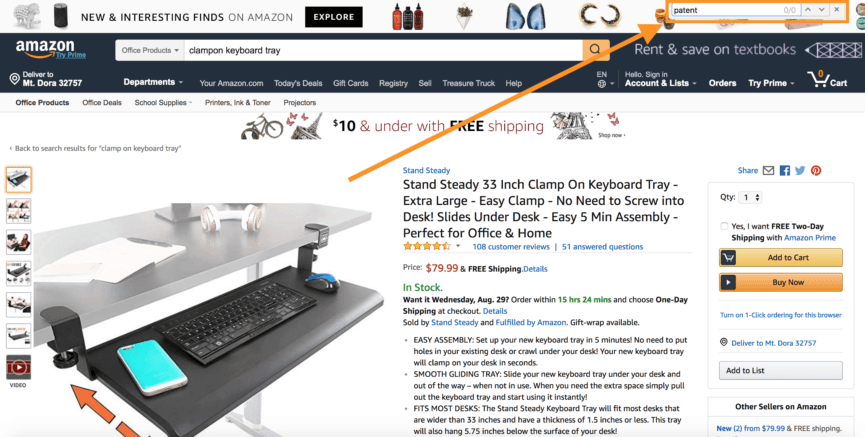This detailed caption describes an Amazon.com product page for the Stand Steady 33-inch Clamp-on Keyboard Tray. 

The screenshot showcases the product aimed at enhancing office ergonomics with its extra-large, easy-to-install design. The tray, titled “Stand Steady 33-inch Clamp-on Keyboard Tray - Extra Large, Easy Clamp, No Need to Screw into Desk, Slides Under Desk, Easy 5-Minute Assembly, Perfect for Home and Office,” highlights various key features suitable for both home and office settings.

Featured prominently in the main image, the clamp-on keyboard tray is displayed mounted on a sleek silver table adorned with typical office supplies, emphasizing its practical application. The black tray holds a sample keyboard, mouse, and phone, visually demonstrating its spacious utility. 

The product has a commendable rating of 4.5 stars out of 5 from 108 customer reviews, and 51 answered questions. It is currently available for $79.99, with stock ready for purchase. The right side of the page provides purchasing options, including buttons for "Add to Cart," "Buy Now," and "Add to List," along with options for sharing, adjusting quantity, checking for used options, and exploring other sellers.

Additional minimized preview images located on the left side can be enlarged to provide further product perspectives.